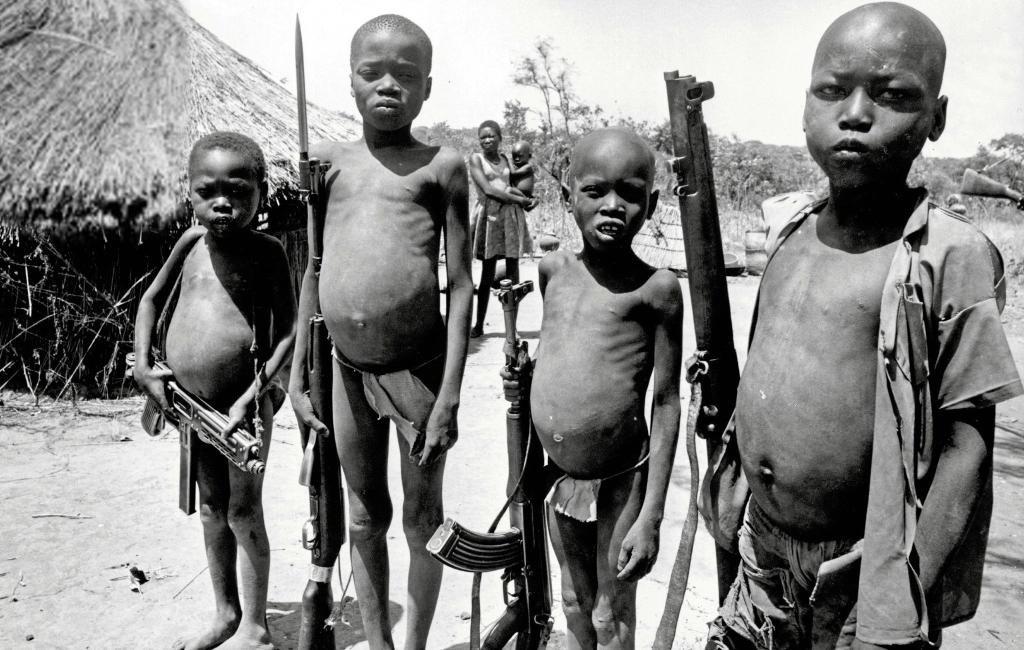This black-and-white photograph powerfully captures the troubling reality of child soldiers in Africa. In the foreground stand four young black children, their bald heads and distended bellies indicative of severe malnourishment or starvation. They are minimally clothed, with three wearing only loincloths while one also dons an overshirt. Each child holds a different type of firearm with a solemn and serious expression directed at the camera: the first child grips a small machine gun, the second wields a rifle with a bayonet, the third clutches an AK-47 with its distinctive curved magazine, and the fourth carries a larger rifle. Their stark presence contrasts sharply with the background, where a village scene unfolds. A grass hut is visible in the upper-left corner, while a woman in a dress, holding a baby, stands amidst sparse, non-plush grass and a scrawny tree, preoccupied with her own concerns. This haunting image underscores the grim circumstances and complex dynamics of life in a conflict zone.